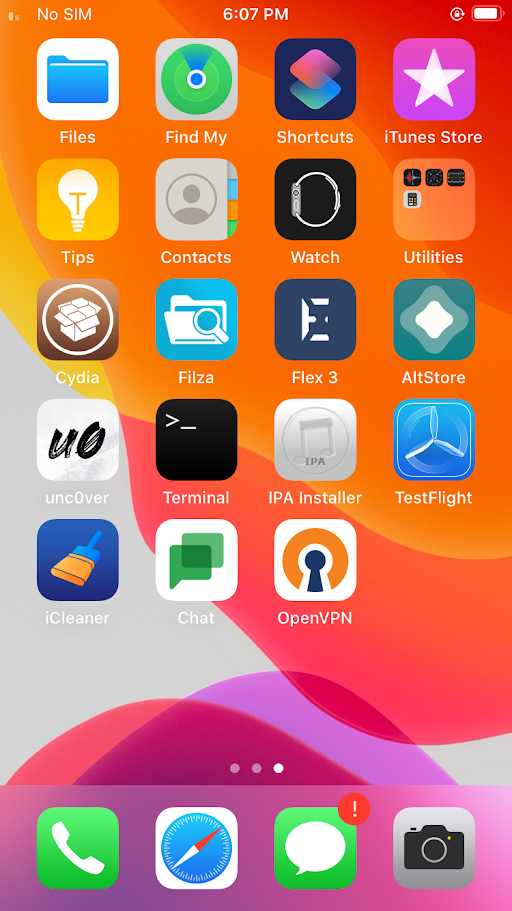The cell phone screen displays a time of 6:07 p.m., with a full battery indicator. The wallpaper features an abstract design with prominent shades of orange, red, gray, purple, and touches of yellow. The top of the screen shows an icon indicating "No SIM."

The home screen is organized into a grid of app icons arranged in multiple rows. The first three rows have five icons each, while the fourth row contains four icons. The apps displayed include:
- Files
- Find My
- Shortcuts
- iTunes Store
- Tips
- Contacts
- Watch
- Utilities
- Cydia
- Filza
- Flex 3
- AltStore
- Unc0ver
- Terminal
- IPA Installer
- TestFlight
- iCleaner
- Chat
- OpenVPN

At the bottom of the screen, the navigation bar features four key icons:
- A green phone handle representing the call function
- A blue and white compass for navigation
- A red circle with an exclamation mark inside a text box, possibly indicating an alert or message
- A camera icon